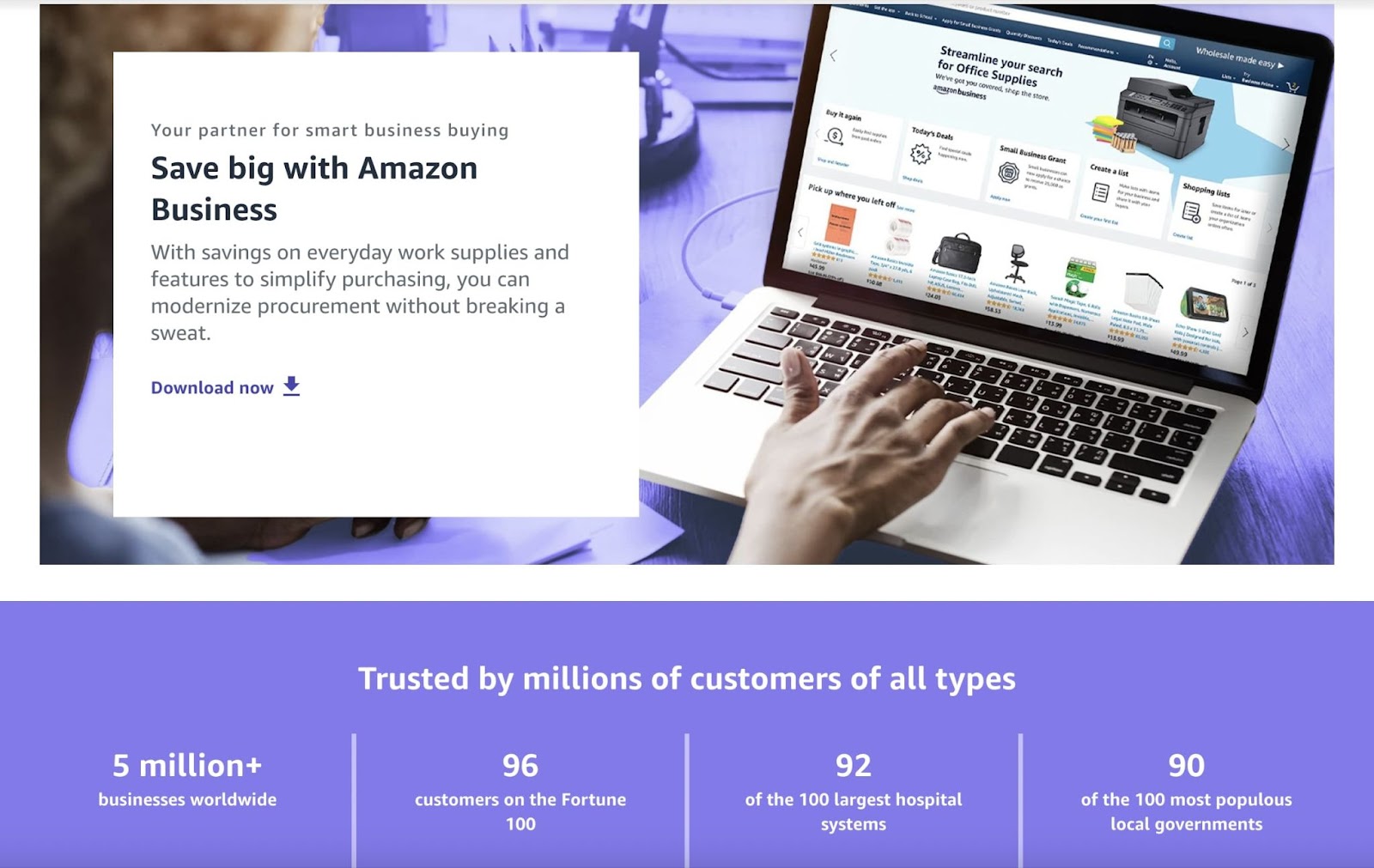This image depicts a web advertisement for Amazon Business set against a blue background. Central to the ad is a person typing on a laptop with their right hand. The screen of the laptop displays a computer-related website, though the specifics are indistinct. The individual in the image has their face partially obscured and blurred by the ad’s design elements.

The primary text of the ad reads: "Your partner for smart business buying. Save Big with Amazon Business." Below, a detailed statistic box in a gradient of light blue and light purple showcases Amazon Business's credibility and extensive reach. It states that the service is trusted by over 5 million businesses worldwide, includes 96 out of the Fortune 100 customers, partners with 92 of the 100 largest hospital systems, and serves 90 of the 100 most populous local governments.